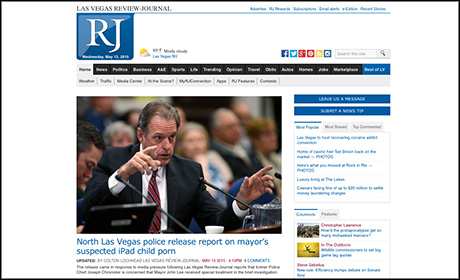The image captures the front page of the Las Vegas Review Journal. In the upper left corner, the text "Las Vegas Review Journal" is prominently displayed. Just below this title is a large blue box with bold white letters "RJ" inside it. Beneath this box, though the text is blurry, one can decipher the word "Wednesday" and potentially "May," along with an illegible date and year. Adjacent to this is an icon of a sun and a cloud, indicating the weather forecast with blurry figures but clearly showing "mostly cloudy" with the temperature in Fahrenheit, specific to Las Vegas, Nevada.

Immediately below this section is a black border containing out-of-focus text, making it largely illegible. However, discernible words include "News," "Politics," "A&E," and "Life." Following this section, a gray background features more options, among which "Contents" is the only recognizable word due to the blurriness of the rest.

The central content of the page is dominated by a large photograph of a man in a suit with a blue and red striped tie. He is seated at a table with microphones in front of him. Several individuals are seated behind him; however, they remain out of focus. The caption for the photograph reads, "North Las Vegas police released report on near suspected iPad child porn."

The right column contains additional text, which is difficult to read, featuring several headlines. The "What's Popular" tab—or possibly "Most Popular"—is highlighted, listing various unreadable headlines beneath it.